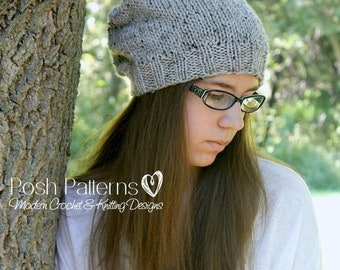The image features a teenage girl with long, cascading brown hair, which flows over the front of her light white shirt, obscuring most of it. She is leaning against a tree positioned to the left side of the frame. The girl is adorned in a knit gray cap and wears dark-framed glasses, her gaze directed downward, lending a contemplative air to her expression. The composition captures her from approximately the shoulders up. The background is a soft blur of leaves and trees, providing a natural, serene backdrop. Superimposed on the image, in elegant white print, the words "Posh Patterns" arc across the tree and her hair, accompanied by a small heart symbol. Beneath this, the phrase "Modern Crochet and Knitting Designs" is also displayed in white, completing the visual narrative with a sophisticated touch.